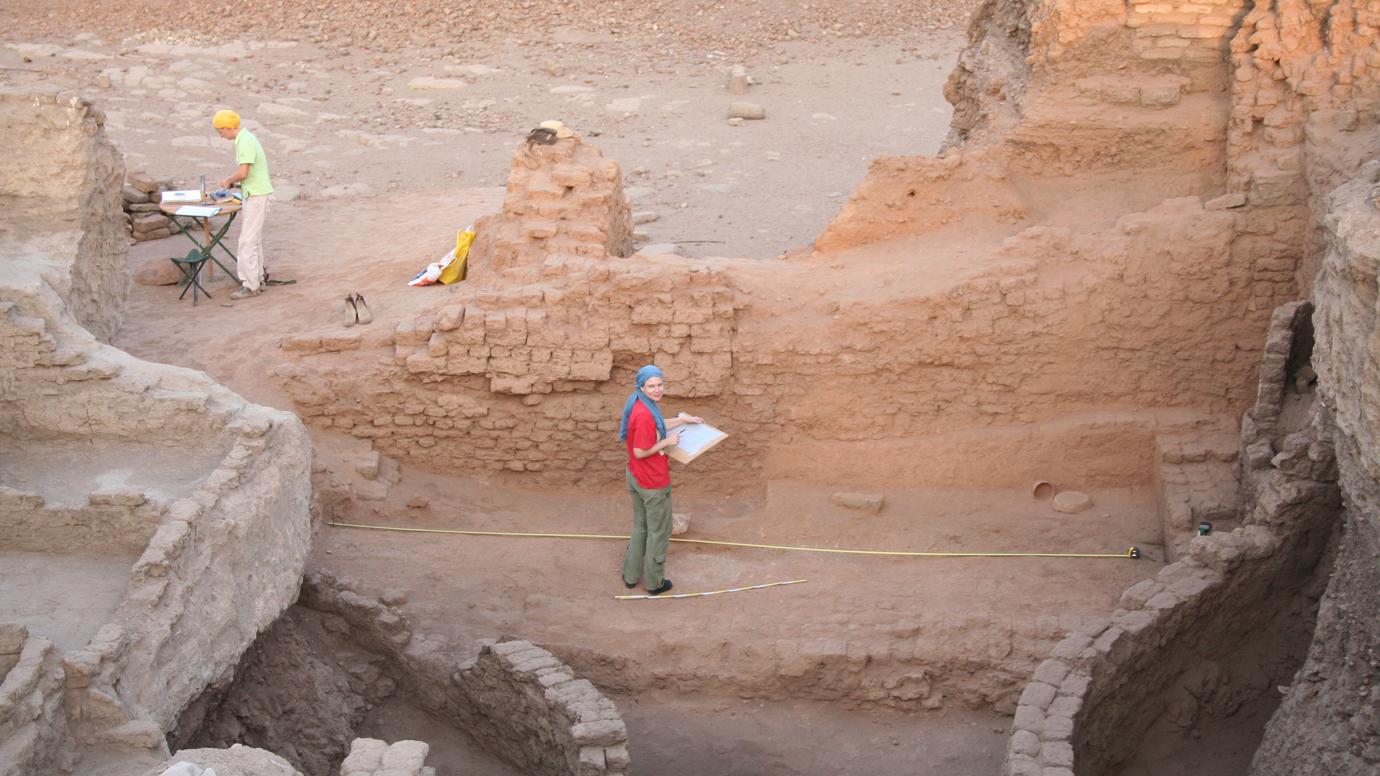The photograph captures an outdoor scene, likely situated at an archaeological dig site within a desert. The environment is characterized by a crevice amid a landscape of sandy rocks, dirt, and remnants of a fallen, reddish-hued brick structure. The broken walls, partially composed of stone and possibly concrete, indicate where rooms might have been in a bygone era.

Two individuals are engaged in activities at the site. Centrally located in the image is a man dressed in a red short-sleeved shirt, olive green pants, and a blue scarf on his head. He holds a clipboard in his hand and is looking towards the camera. Approximately 10 feet to his left, another man stands at a portable table, covered with scattered papers, giving the appearance of a makeshift desk. This second man sports a very light green shirt, white pants, and a yellow cap, with a yellow item that resembles a backpack placed beside or behind him.

The ground is strewn with dirt, and a sandy rock wall encircles the scene, creating an enclosed feeling. The sky isn't visible, but the dry condition suggests a clear, nice day without rain.